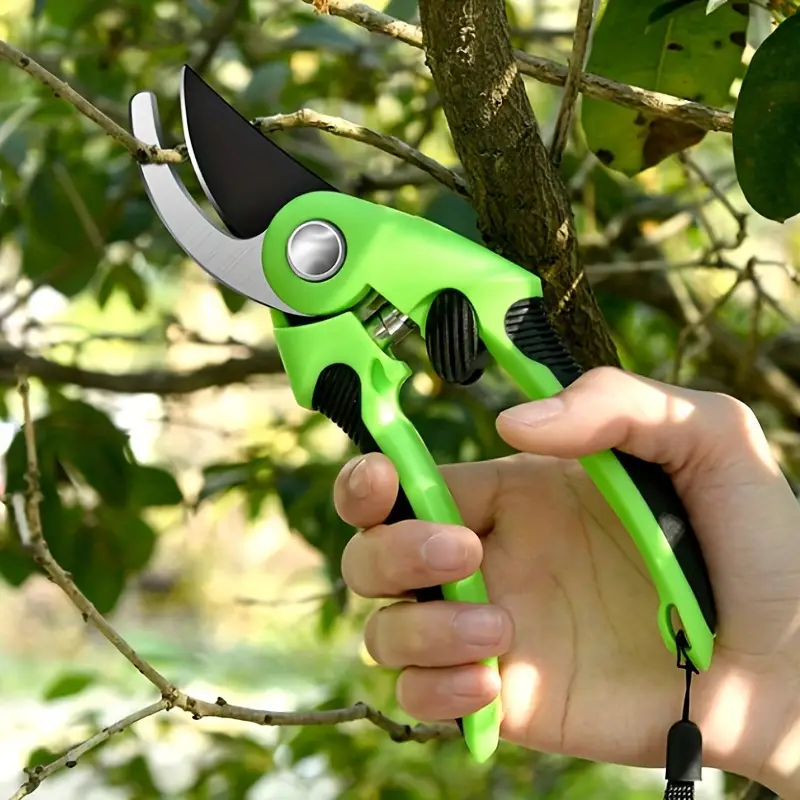This is a detailed, close-up, color photograph in a square format, depicting a hand holding a modern set of pruning shears poised to trim a small branch from a tree. The person's hand, appearing androgynous and likely belonging to someone between 20 and 40 years old, enters the frame from the bottom right, with the palm facing the viewer. The fingers are wrapped around the handles of the shears, which are lime green plastic with black cushioned grips on the top and bottom. A chrome-colored bolt at the top of the handles holds the shears together. The top blade is black with a convex angle, while the lower blade is sharp and silver, both surrounding a small twig, ready to cut. In the blurred background, a tree trunk with various branches and dark green foliage provides a contextual setting for the pruning activity.